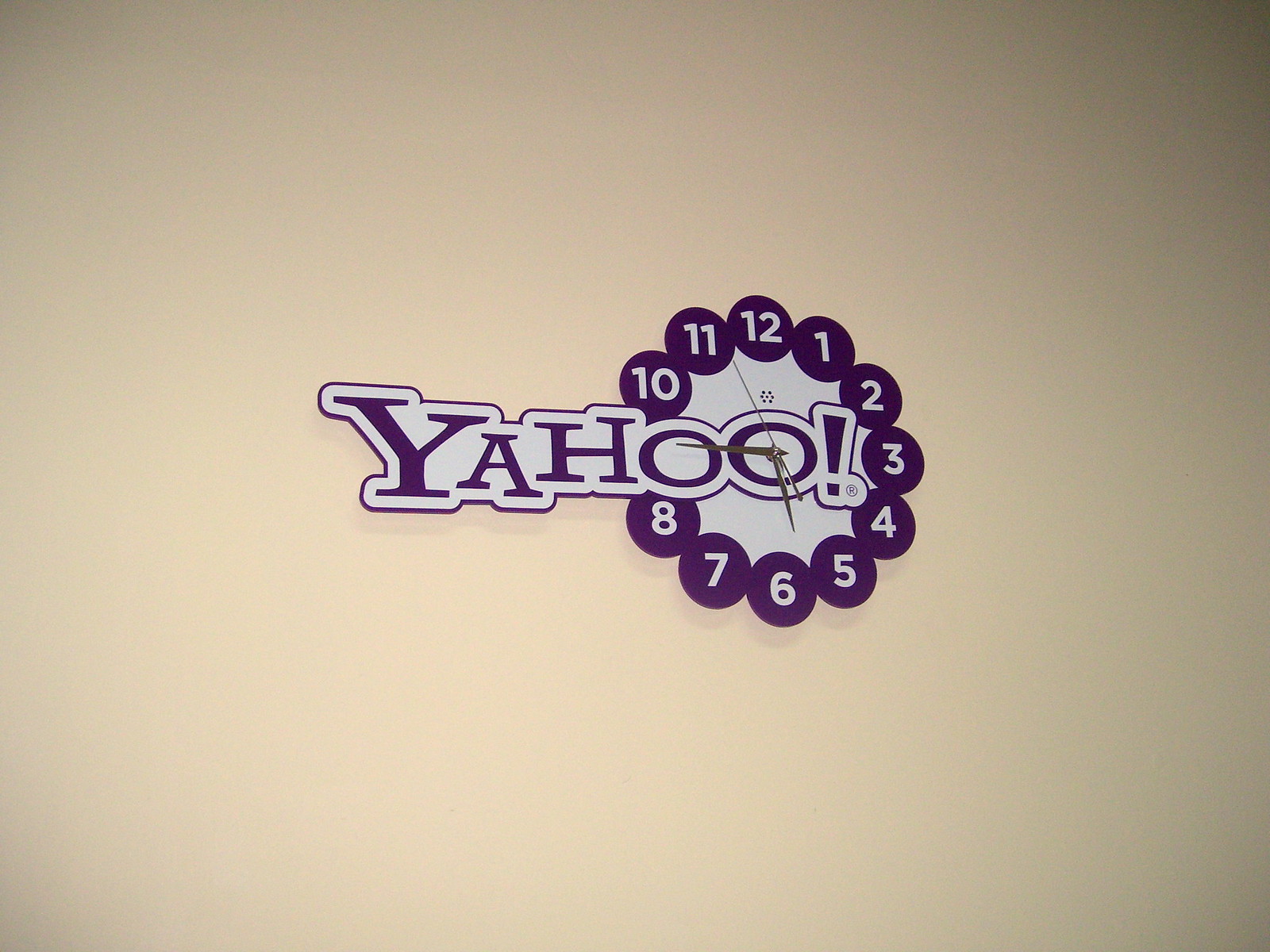In the image, a pristine white wall serves as the backdrop. Prominently featured in the middle is the word "YAHOO" rendered in bold, purple lettering. Surrounding the central text, there are numbers ranging from 1 to 12, arranged in a circular pattern reminiscent of a clock face. Within this circle, there is another smaller white circle containing several dots that suggest a speaker or a focal point. Some hands within the circle are specifically pointing towards the number 11, while our hands are extended towards the left, directing attention across the "YAHOO" inscription. The purple letters of "YAHOO" are further accentuated by a subtle white outline. Additionally, there are purple circles with white text inside positioned around the scene, adding to the visual arrangement.